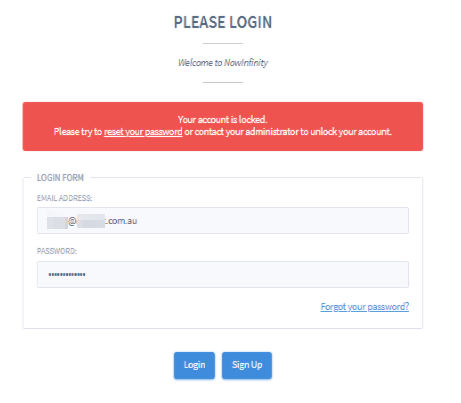The image depicts a login page with a structured and clean design. At the top, on a white background, there is a bold, gray-colored text that reads "Please Log In." A thin gray line runs horizontally beneath this text, visually separating it from the next section. Following this, you see the phrase "Welcome to NowInfinity," where "NowInfinity" is presented as a single word in a thinner typeface compared to the "Please Log In" heading. Another thin gray line is placed under this welcome message, further dividing the sections. 

Below these lines, a bold red rectangular box with white text inside alerts the user that their account is locked. The message reads: "Your account is locked. Please try to reset your password or contact your administrator to unlock your account." The phrase "Reset your password" is underlined for emphasis.

Underneath this alert, gray-colored text states "Login Form," which is accompanied by a gray rectangular outline that frames input fields for the email address and password. A blue "Forgot Your Password" link is positioned at the bottom right of this section. Finally, at the bottom of the page, there are blue "Login" and "Setup" buttons available for user interaction.